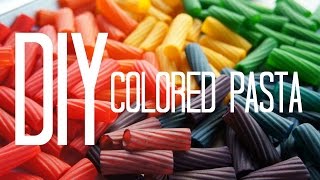The image showcases a variety of vibrantly colored pasta, possibly ziti or rigatoni, arranged haphazardly on a plate or in a shallow dish. The pasta colors range from red, orange, yellow, green, and purple to nearly black. The pieces are scattered randomly, with some lying horizontally, others vertically, and some slanted, creating a chaotic yet colorful display. Overlaid on the image is an imposing text in white, capital letters reading "DIY" in large font, followed by "colored pasta" in significantly smaller but still uppercase letters. This text reinforces the do-it-yourself theme of the colorful pasta presentation.